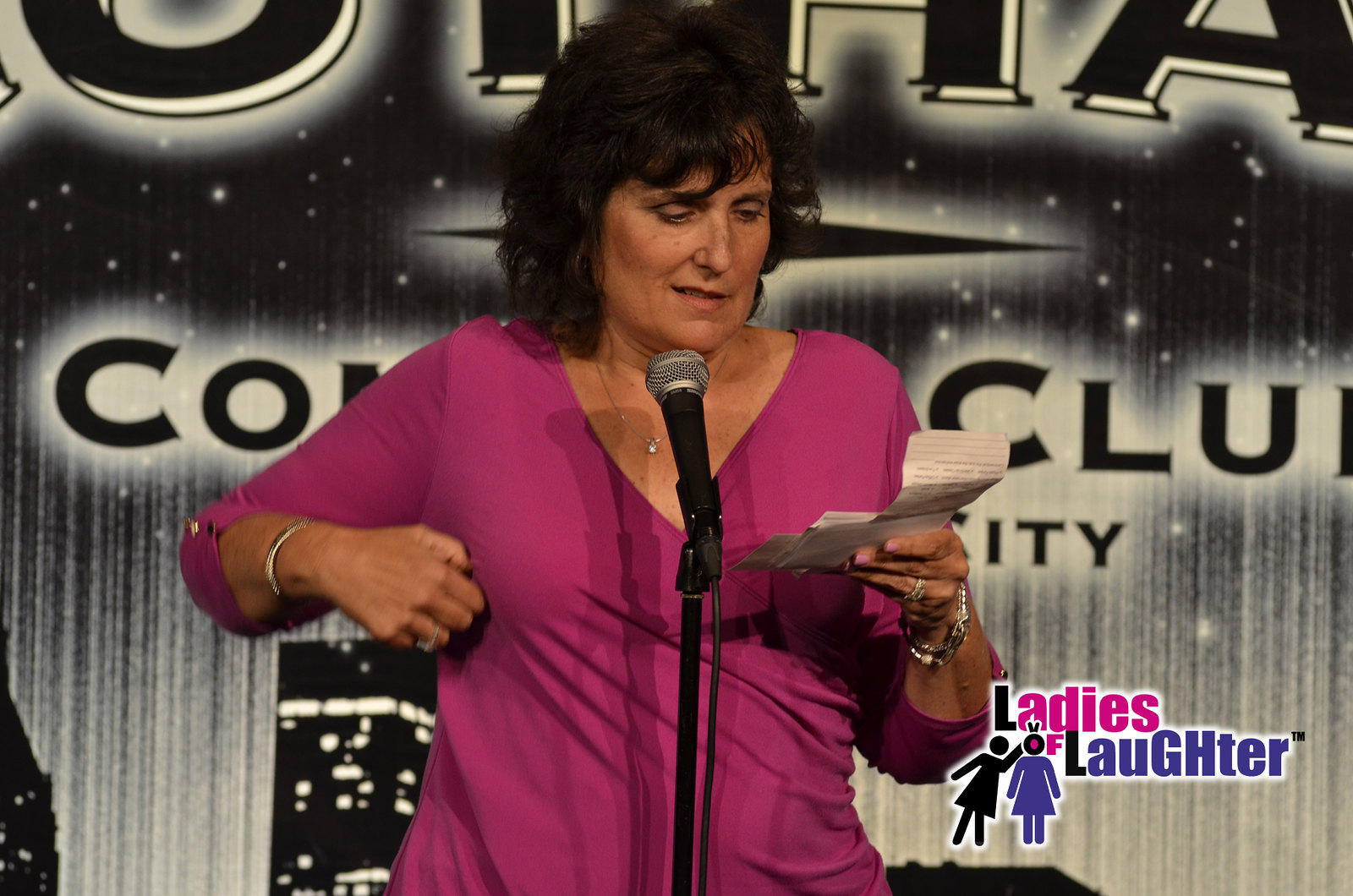The image depicts a woman with shoulder-length curly black hair and dark eyebrows, wearing a long-sleeved, pinkish-red V-neck shirt. She is standing on stage with a microphone, reading from several small pieces of paper in her left hand. She has a thin chain necklace with a clear stone around her neck, a silver bracelet on her right wrist, and additional bracelets on her left wrist, as well as a ring on her ring finger. The backdrop includes a black, white, and grey cityscape with stars and skyscrapers, and partially visible large black letters that cannot be completely read. In the bottom right corner, there is an emblem with the text "Ladies of Laughter" in pink, blue, and black, accompanied by outline images of two women, one appearing to touch the other's head, forming the word "of" in the title. The woman appears to be scratching her armpit with her right hand while focusing on the papers she is reading.